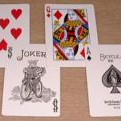A small photograph captures a sequence of playing cards meticulously arranged on a brown carpet. The spread includes the Six of Hearts, a Joker, the Queen of Hearts, and the Ace of Spades. The composition of the image and the close-up perspective draw attention to the intricate details of each card set against the textured carpet background.